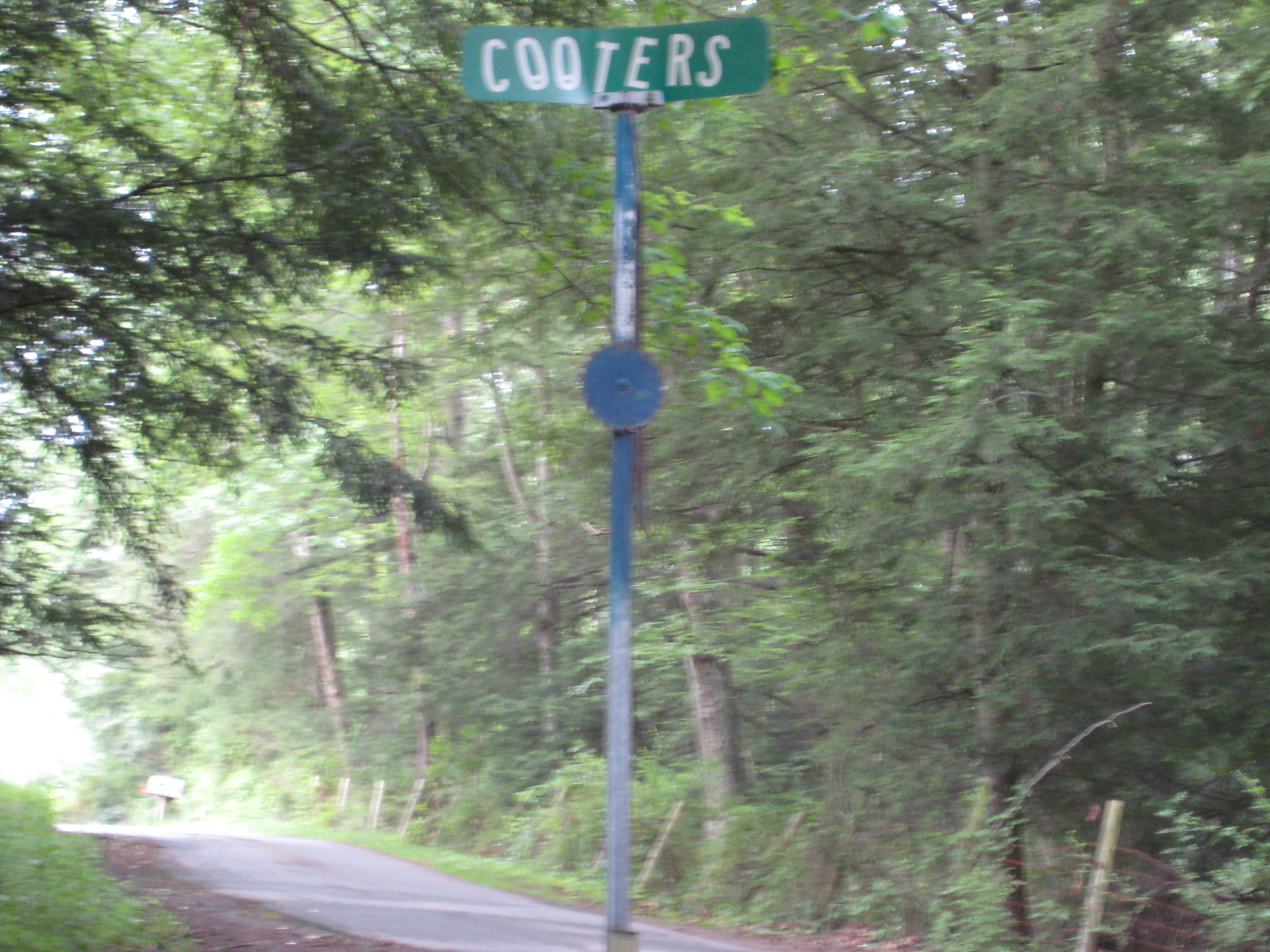In this slightly horizontally rectangular outdoor image, natural lighting illuminates a densely wooded backdrop with trees in various vibrant shades of green. From the bottom center extending diagonally to the lower left corner, a narrow, paved single-lane road meanders through the scene, evoking a quintessential rural ambiance. Dominating the center of the frame and nearly reaching the top, a large metal signpost stands tall. The signpost is predominantly metal gray, with a notable blue circle mid-height that adds a touch of color contrast. Affixed to the very top of the post is a horizontally rectangular green street sign, which appears to be handcrafted. In white letters, it reads "Cooters," with the two O's artistically depicted as eyes gazing downward, adding a whimsical and personalized touch to the rustic setting.